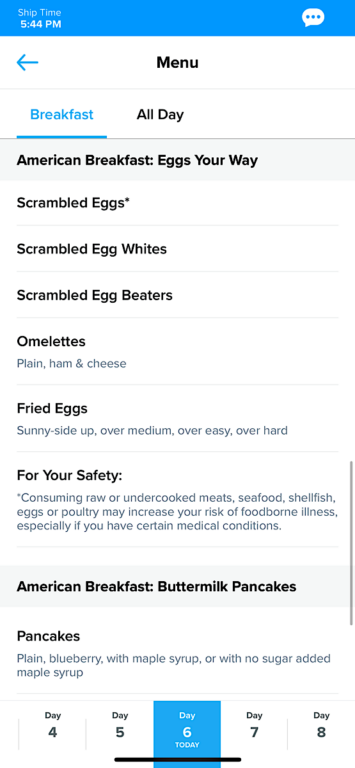The image on an Apple device displays a food ordering app, specifically highlighting the breakfast menu. At the bottom, there's a horizontal bar for exiting the app. The screen has a medium blue rectangle across the top with white text stating "Ship time 5:44 PM" accompanied by a small chat bubble icon with dots inside. A blue left-pointing arrow and the word "Menu" in black text are also visible at the top.

Currently, the "Breakfast" section is highlighted with blue text and an underline. Another visible option is "All Day." The menu lists various breakfast choices, some with detailed descriptions. The options include:

- American breakfast
- Eggs your way:
  - Scrambled eggs (with an asterisk)
  - Scrambled egg whites
  - Scrambled egg beaters
- Omelettes (description: plain, ham, and cheese)
- Fried eggs:
  - Sunny side up
  - Over medium
  - Over easy
  - Over hard

There is a safety disclaimer noting that consuming raw or undercooked meats, seafood, shellfish, eggs, or poultry may increase the risk of foodborne illness, especially for individuals with certain medical conditions.

The menu transitions to a new section for American breakfast buttermilk pancakes, offering options like plain pancakes, blueberry pancakes, with maple syrup, or with no sugar added maple syrup.

The bottom part of the screen allows users to select the delivery date, showing options with days labeled from four to eight. "Today" is highlighted in blue with white text, while the other days have a white background and black text.

The image suggests the app is being used to order breakfast for delivery.